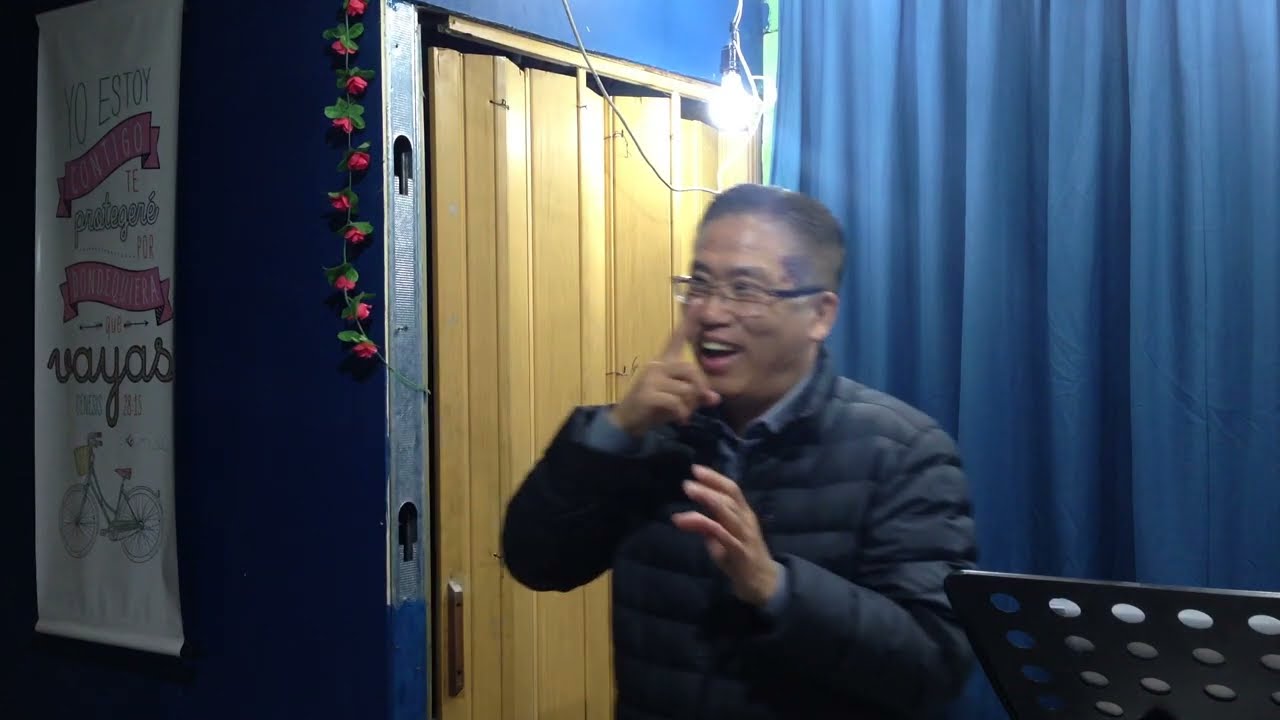The image features an Asian man with short, slightly graying hair, wearing glasses and a dark blue puffer jacket over a blue shirt. He stands in the center, slightly to the right, with both hands raised - his right hand touching his nose and the left one extended outward. The man appears to be laughing. Directly above him, a light bulb hangs, illuminating the scene. To his left, a brown sliding door is visible, and to its left, a white sign with pink and green accents reads "Yo estoy contigo" with a small drawing of a bicycle at the bottom. Between the sign and the door, a hanging plant with budding flowers adds some greenery. To the man’s right, there's a black sheet music stand and behind him, blue curtains form the backdrop. The setting seems to be indoors, possibly in a studio.